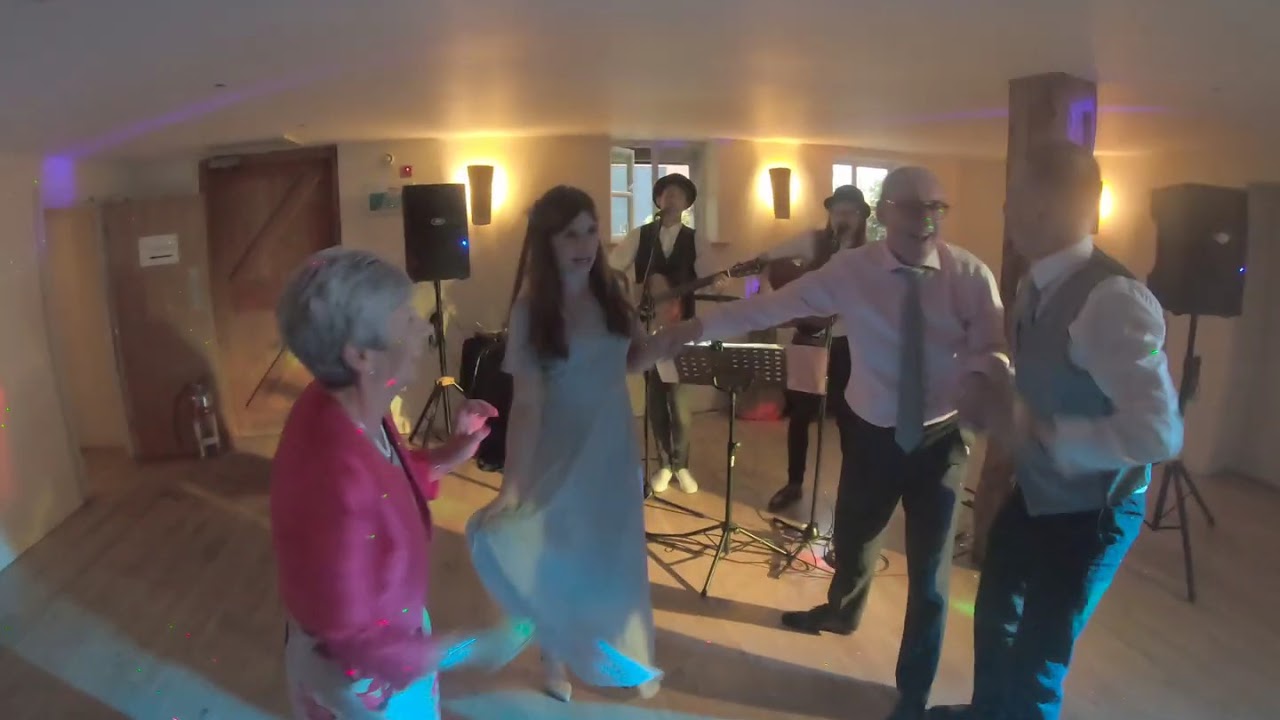In this indoor, dimly lit scene, possibly a party or rehearsal in a basement recreation room, several elements catch the eye. The image is blurry and dark, with a low white ceiling, wooden floors, and walls adorned with soft wall sconces. Bright light floods in through basement windows, creating stark contrasts but failing to adequately illuminate the room. 

Central to the background are two musicians wearing matching outfits of long-sleeved white shirts, black vests, pants, and hats, stationed in front of microphones, music stands, and amplifiers. They appear to be playing guitars, though details are obscured due to the poor lighting and blurriness.

In the forefront, four people stand, possibly dancing or mid-conversation. On the right, a middle-aged, bald man wearing glasses, a white shirt, blue tie, and dark pants smiles as he engages a younger man in a blue vest, white shirt, and dark pants. Their proximity suggests they might be talking or exchanging a jovial moment.

Near the center of the group, a young woman with long brown hair, dressed in a soft, floaty, floor-length blue dress, holds up her skirt as if preparing to dance. She grasps the hand of the bald man, indicating a possible dance move or a shared merriment. 

Flanking the group on the left is an older woman with silvery short gray hair, adorned in a pink sparkly jacket over a blue floral skirt, accessorized with pearls around her neck. Her stance and gesturing suggest she may be contributing to a lively discussion or addressing the group.

The color palette of the scene is predominantly sandy tan for the environment, with clothing hues of pink, blue, white, and black adding visual interest despite the overall lack of focus and clarity in the image.